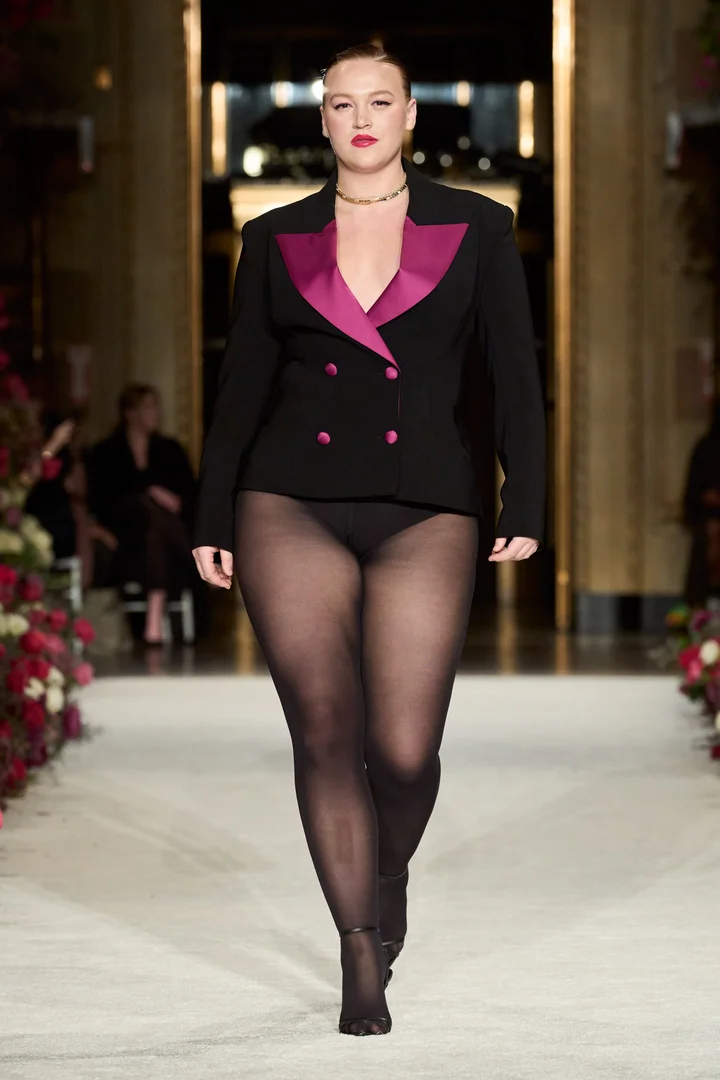This photograph showcases a plus-size model confidently walking down a white runway, which is adorned with multicolored roses in red, white, and pink along the edges. She is front and center in the image, with a slightly blurred background focusing all attention on her. The model is wearing a tailored black jacket with striking fuchsia pink lapels and four buttons arranged in the corners of a square beneath the lapels. The jacket stops at her hips, revealing black underpants and sheer black pantyhose. She is barefoot, her feet covered only by the pantyhose. Her hair is pulled back tightly, enhancing her facial features, and she sports a gold choker around her neck, minimal makeup, and bold red lipstick. The background features a brown wall with a prominent gold doorway, and there are spectators slightly visible, seated and watching the runway show.